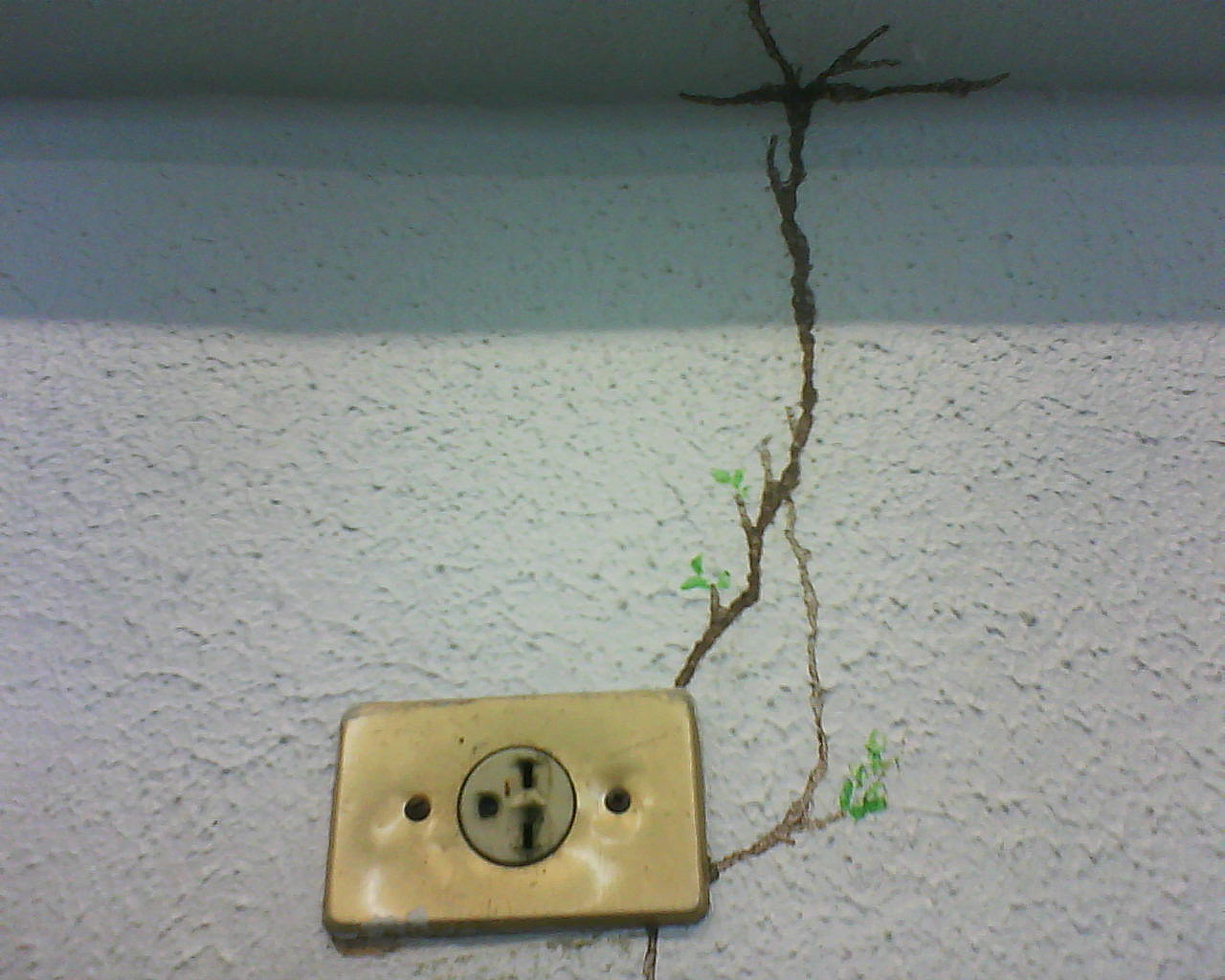The photograph showcases an old, uniquely designed electrical outlet mounted on a white, rough-textured wall that extends up to the similarly textured ceiling. Unlike standard outlets, this one has a single circular socket at its center, framed by a rectangular, shiny gold or bronze metal casing secured with screws. The outlet itself has scorch marks around its edges, suggesting wear over time. Intriguingly, there is an artistic element painted on the wall: a brown vine with a few small green leaves appears to grow out from the outlet, extending upwards and across the ceiling. The painted vine cleverly mimics a real plant, blending art with functional elements in an eye-catching manner. Sunlight casts shadows on the textured wall, adding depth to the scene while highlighting the unique interplay between the outlet and the painted vine.